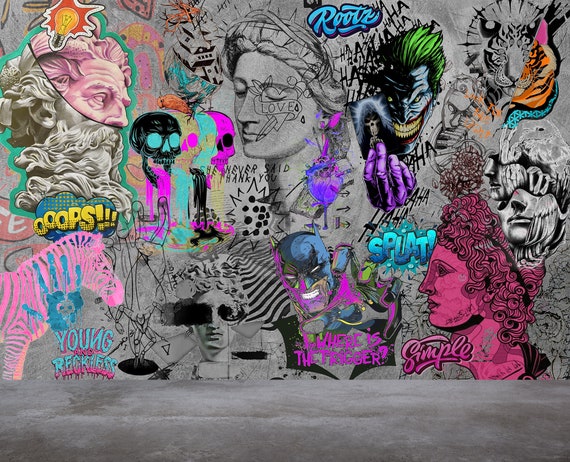The image depicts an intricate, digitally-stylized graffiti mural on a gray cement wall with a gray cement floor. The vibrant and eclectic artwork features a blend of ancient Grecian busts and modern pop culture icons. Prominent among the figures are a realistic depiction of the Joker from Batman, Batman himself, a half-pink, half-marble Grecian statue, and the Statue of Liberty's head in the center. Scattered throughout the mural are neon-colored elements including a bright pink zebra with a blue handprint across it, and various skulls painted in black, yellow, blue, and hot pink. Words and phrases like "Young Reckless," "Oops," "She Never Said Thank You," "Roots," "Splat," and "Simple" are tagged in assorted colors and fonts. Additional details include a tiger that is half colored and half black and white, and a face with curly purple hair and a purple face. The mural is a busy mosaic of individual pieces, creating an overall larger and vibrant street art fresco.